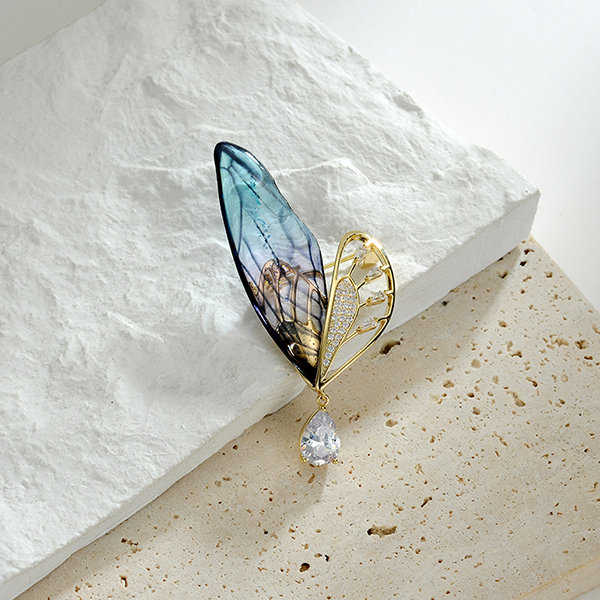The image features a close-up color photograph of a butterfly-shaped necklace with one wing crafted from gold, possibly embedded with tiny diamonds or sparkling stones, and the other wing designed to resemble a real butterfly, potentially made from glass. Below the wings hangs a sizable teardrop-shaped clear gemstone, which could be a cubic zirconium or a similarly faceted white gem. The jewelry rests on a piece of white styrofoam, which is positioned on top of a white, flat rock-like surface with small holes, against a white background. The overall setting gives an impression of elegance and luxury.